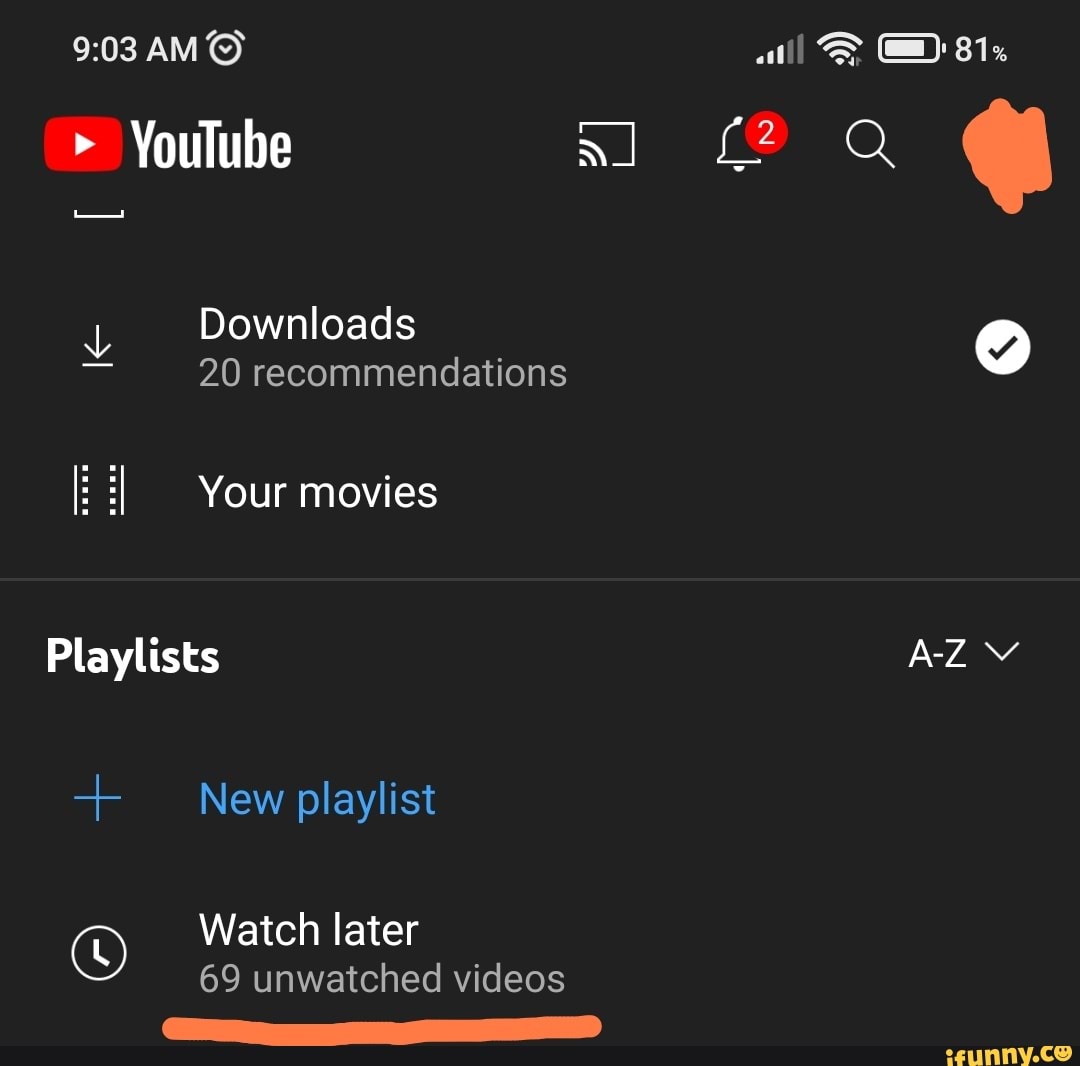The image depicts a phone screen displaying a YouTube page with a predominantly black background and white text. In the top left corner, the time reads "9:03 AM" accompanied by an alarm clock icon. The top right corner features icons indicating cellular connection, a wireless symbol, and a battery icon showing 81% charge.

Centered below these icons is the YouTube logo followed by the word "YouTube." Directly underneath, there is a downward-pointing arrow and a horizontal line separating this section from the next. It reads "Downloads, 20 Recommendations," with a white circle containing a black check mark situated to the right.

Further down, a segment labeled "Your Movies" is in white text next to a small film reel icon. Adjacent to this is the bolder label "Playlist." Opposite is a "A to Z" label with a downward-pointing arrow next to it. Below this, a blue plus sign is followed by the blue text "New Playlist."

In the lower section, there is an icon of a clock with clock hands inside a circle. To the right, it reads "Watch Later" in white text, with "69 Unwatched Videos" written in slightly smaller white text beneath it. An orange, hand-drawn line underlines "69 Unwatched Videos," adding a pop of color to the otherwise monochromatic scheme.